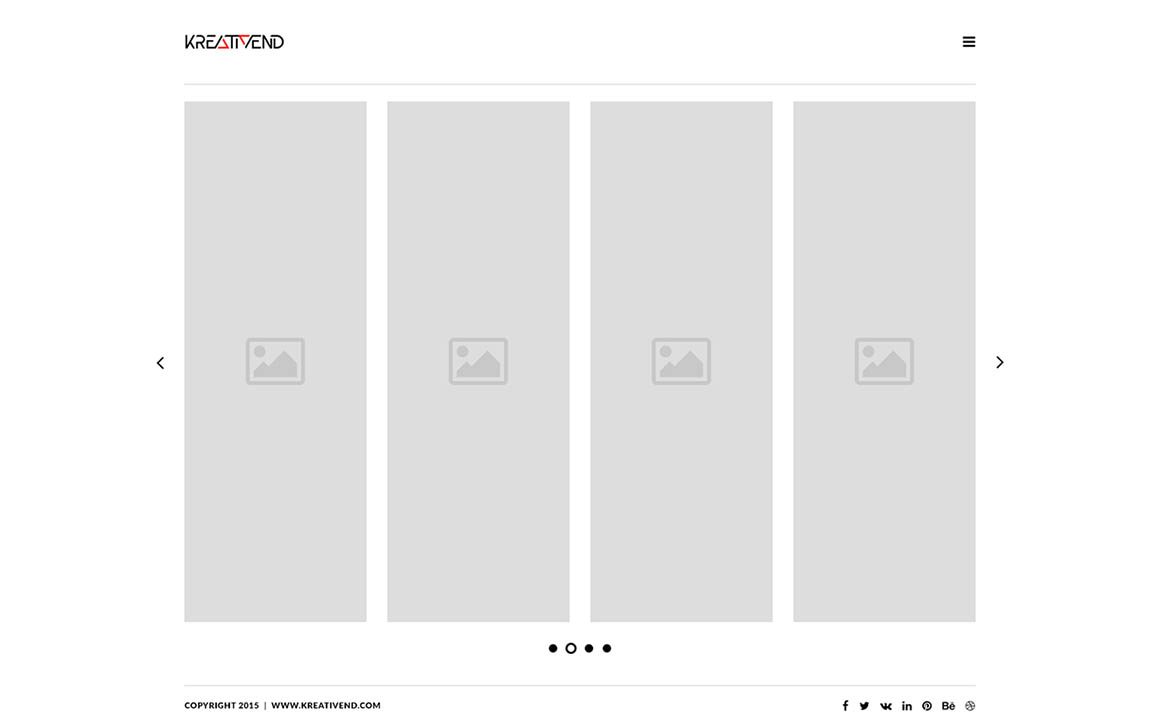This image is a minimalist screenshot from a digital interface, possibly from a computer or smartphone. The upper left corner features the text 'KREATIVEND' in a distinctive font against a white background. Directly below this text, there are four narrow vertical gray rectangles in a row, each separated by a small white space. These rectangles contain placeholder icons of a small square with a mountain and sun, suggesting that these are slots where images can be uploaded or dragged and dropped.

Toward the bottom of the image, there are four black dots arranged horizontally in the lower center, indicating that the user is on the second page of a multi-page interface. In the bottom right corner, small text reads 'Copyright 2015 www.creativen.com'. Alongside this text, there are icons for popular social media platforms such as Facebook, Twitter, and Instagram, providing easy access for sharing or connecting through these networks.